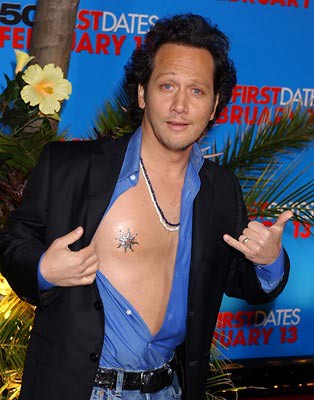The image features a close-up of a man with wavy black hair and blue eyes, positioned centrally in the frame. He has olive-colored skin and is dressed in a royal blue collared shirt, which is unbuttoned, revealing a star-shaped nipple cover on his chest. Over the shirt, he wears a black suit jacket and accessorizes with two necklaces, one light and one dark. His attire is completed with blue jeans and a dark belt. The man is standing in front of a blue wall, which has the text "50 First Dates" and "February 13th" written in red. The background also includes decorative elements such as a yellow flower and what appears to be a green palm tree design. He is making a gesture with his hand, extending his thumb and little finger.